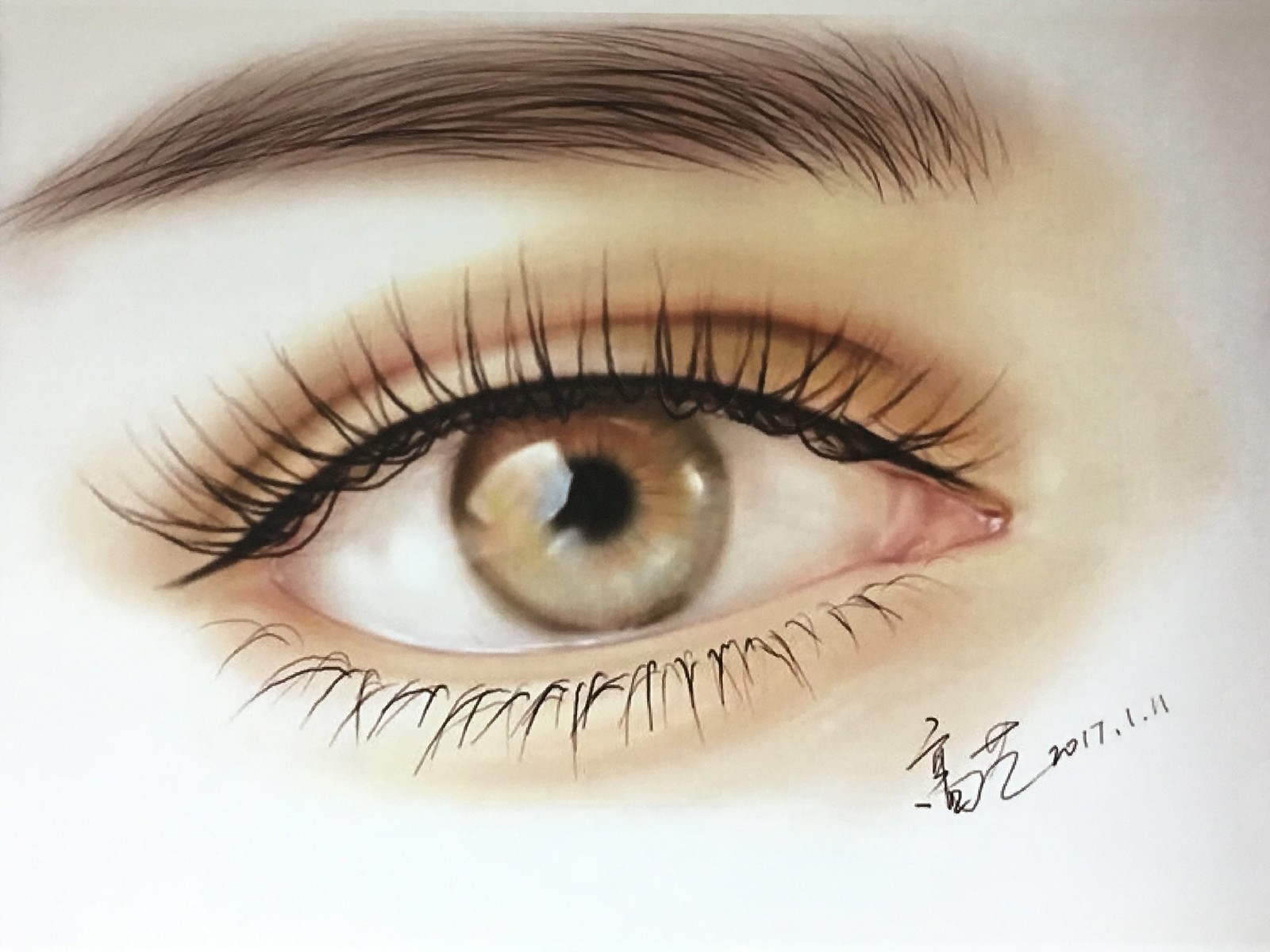This is a detailed, color illustration of a woman's right eye, rendered with near-photorealistic precision. Set against a white backdrop, the top left and right corners gradient into grey, adding a subtle contrast. The eye itself possesses a captivating hazel hue, blending light brown with shades of green. There is a meticulous reflection captured within the eye, enhancing the lifelike quality of the artwork. The upper lashes, coated in mascara, frame the eye with thick, black strokes, while the bottom lashes provide a delicate balance. The inner corner of the eye is depicted in a natural pink tone, contributing to the realism. Above the eye, the eyebrow is detailed in brown, matching the overall color scheme. A layer of light brown eyeshadow decorates both the upper and lower eyelids, intensifying in shade near the upper inner corner, right above the pink tear duct. The artist's signature, dated 2017, features prominently in the bottom right corner, marked with a unique "1/1" notation, signifying perhaps an exclusive work.